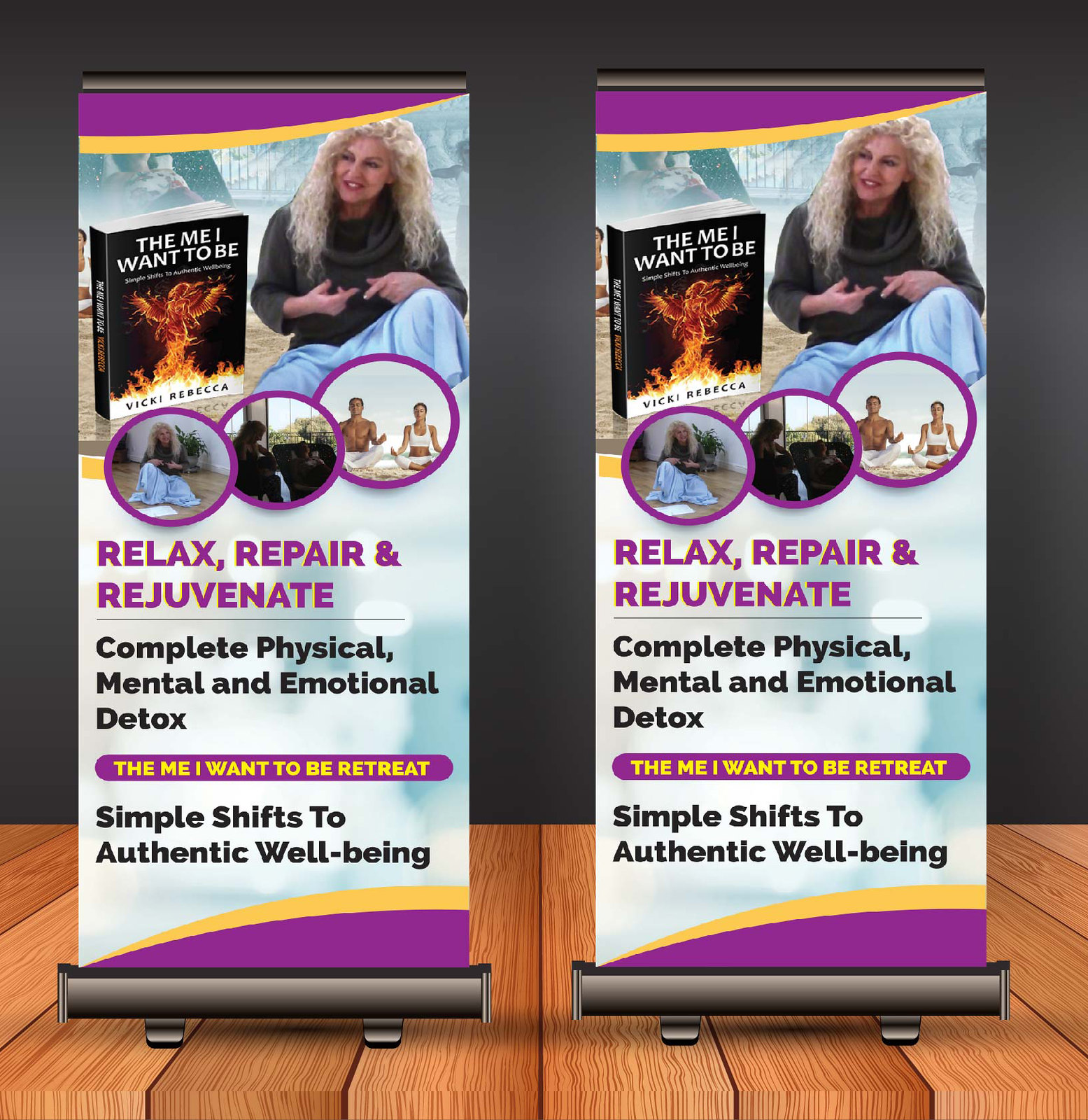The image depicts two identical floor-standing banners positioned side by side on a wooden floor with a black wall in the background. Each banner features a prominent image of a woman with curly blonde hair at the top, adjacent to a large depiction of her book titled "The Me I Want to Be" by Vicki Rebecca. The book cover includes an intriguing, flaming figure that might represent a woman with wings. Below this visual, three circular insets showcase additional pictures of the author, Vicki Rebecca, including one of her meditating with another person. Underneath these images is purple text stating “Relax, Repair, and Rejuvenate,” followed by black text that reads “Complete Physical, Mental, and Emotional Detox.” The banners also mention "The Me I Want to Be Retreat" and emphasize “Simple Shifts to Authentic Well-Being.”